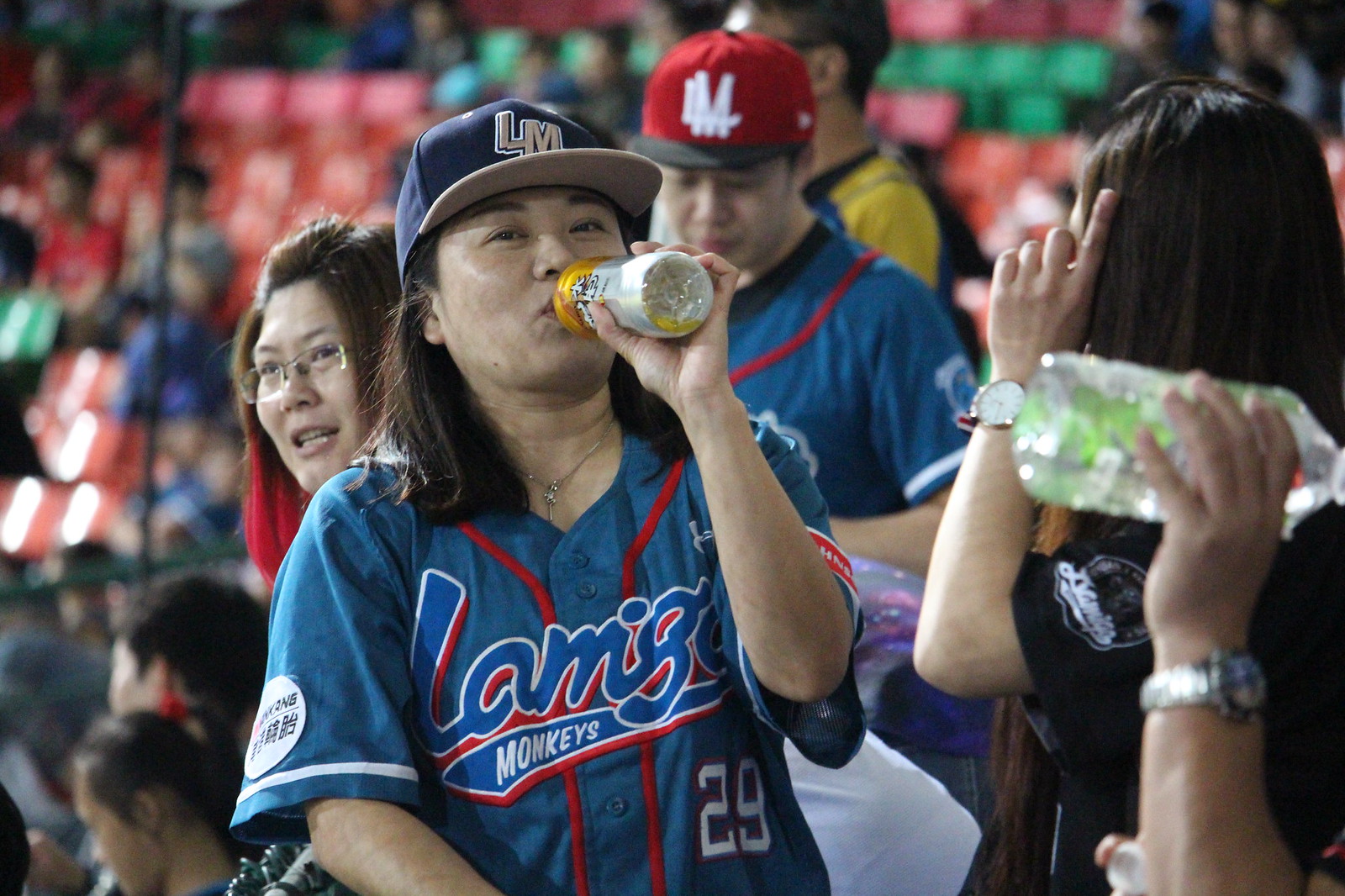Amidst a bustling crowd at a likely Asian baseball stadium, discernible by the vibrant red seats and diverse attendees in the blurred background, the primary focus is a woman in her 30s to 40s. She has shoulder-length, straight dark brown hair and is dressed in a distinctive blue jersey with red accents, suggesting she is either a player or an enthusiastic fan. The jersey partially reads "Monkeys," with the number 29 in white on the bottom right, and she complements her outfit with a matching blue baseball cap emblazoned with "LM." She is captured sipping from a drink with gold and silver packaging, peering directly into the camera amidst the lively, multicolored seating and people surrounding her.